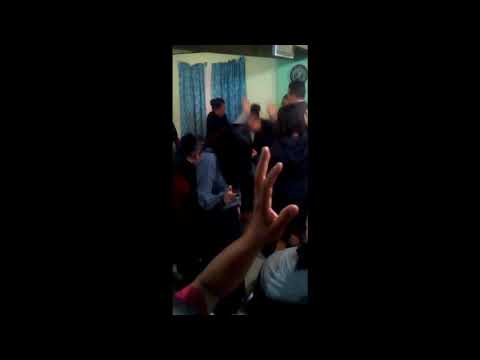The image depicts a gathering of people in what appears to be a small room, possibly a church due to the raised hands suggesting worship or prayer. The room has lime green and darker green walls with blue-teal curtains in the background. Despite the image's low resolution and small size, making it difficult to discern faces clearly, the scene is animated with raised hands and engaged individuals. There are around 10 people visible, with additional people possibly surrounding them. Some participants appear to be older, and a mix of standing and sitting postures is observed. Light streams through the crowd, contributing to the dynamic and lively atmosphere. There is also a round object on one of the walls, adding to the room’s decor.